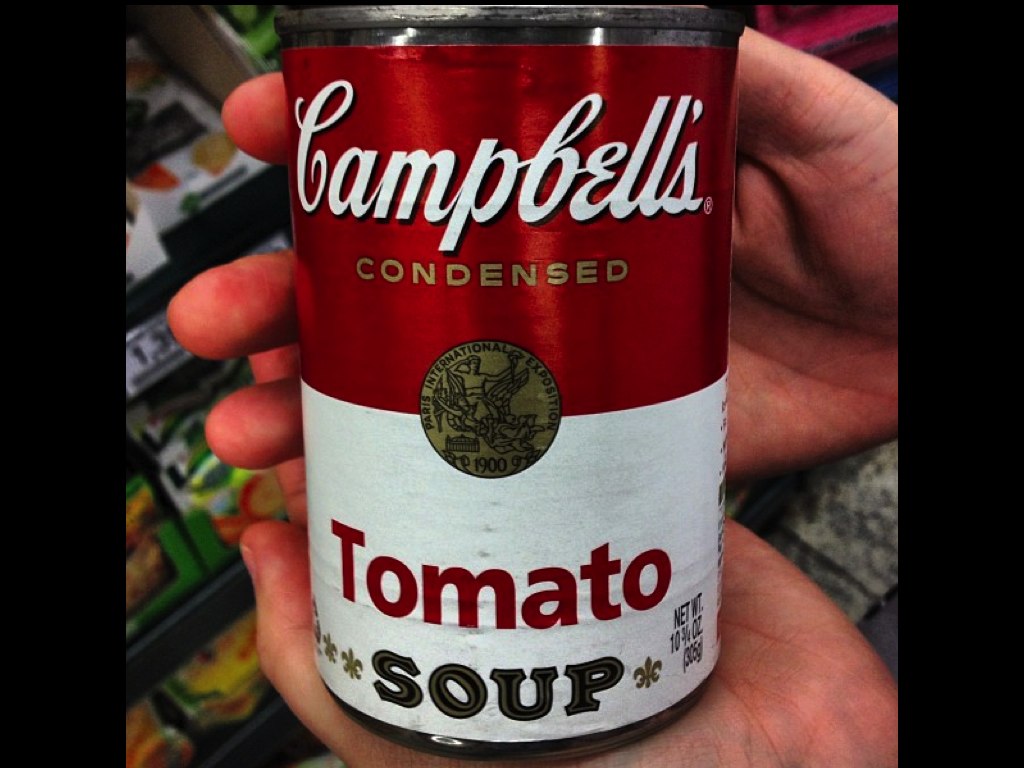In this detailed, close-up photograph, a can of Campbell's condensed tomato soup is prominently displayed, being held by two fair-skinned hands. One hand cradles the bottom of the can, while the other hand supports its back. The upper label of the aluminum can is red, transitioning to white at the bottom. In elegant white cursive font, the name “Campbell’s” stands out at the top, complete with a registered trademark symbol (®). The word "Condensed," in a shade close to gold or bronze, is positioned beneath the brand name. "Tomato," written in bold red letters, is situated in the white section of the label, with "Soup" in a somber gray or black tone just below it. Additionally, there's a small detail in the center of the can proclaiming "International Exposition 1900." The background suggests a supermarket setting, blurred but hinting at other grocery items on the shelves. The net weight of 10 and 3/4 ounces is marked in black lettering, adding to the detailed visuals of this Campbell's soup can.